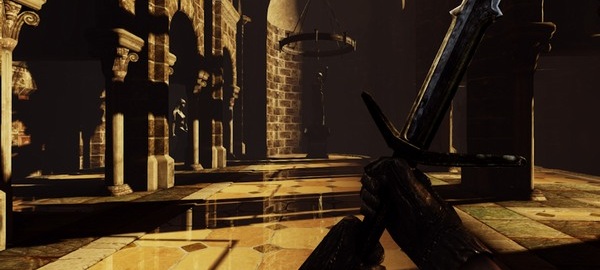The image depicts a dimly lit scene, resembling a medieval castle dungeon, with a focus on brick and tile structures. The setting appears to be a 3D render made in a game engine like Unity or Unreal Engine, viewed from a first-person perspective where the protagonist holds a knife or sword. On the left side, there are several red or brown brick walls and posts, possibly with archways reminiscent of an old fireplace or structural beams. The flooring is a polished surface with intricate tile patterns, featuring rectangular and diamond shapes in shades of brown and tan. There are multiple steps leading up to a higher level in the image. The overall atmosphere is dark, emphasizing the intricate details of the brickwork and flooring more subtly.